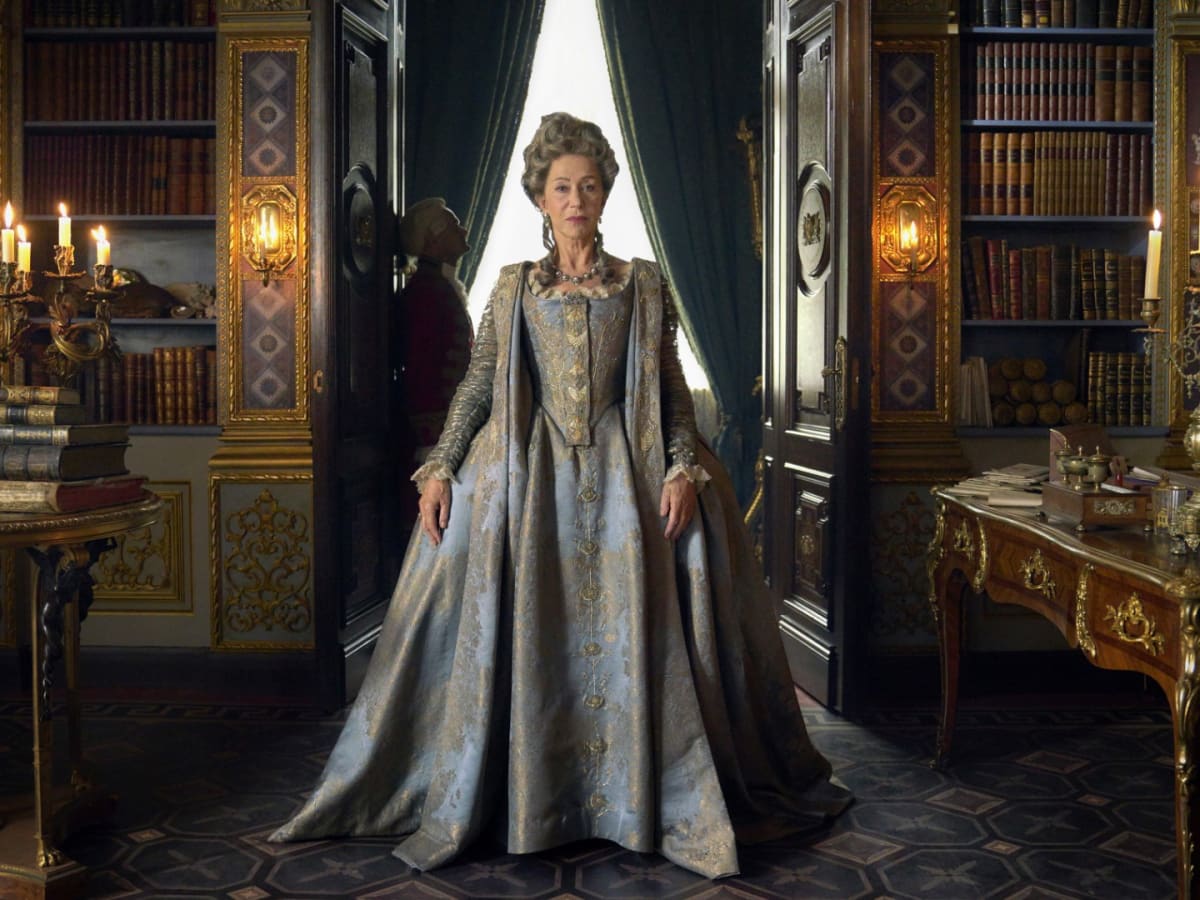The image is a color photograph in landscape orientation, showcasing a middle-aged to older woman, identified as actress Helen Mirren, dressed in a Victorian-era period costume from the film "Catherine the Great." She stands with impeccable posture and a serious expression, facing the viewer. Her luxurious gown is a blend of gold, blue, and lavender with intricate brocade details, complemented by a Victorian-style gray wig intricately curled and piled atop her head. Elegant earrings and a necklace adorn her, enhancing her sophisticated appearance.

Helen Mirren is positioned in front of an ornate doorway with dark brown wood doors, adorned with detailed carvings. Behind her, a man in profile, possibly a butler, holds a brocade curtain open, adding to the historical authenticity of the scene. The room resembles a grand parlor or library in an old mansion, with tall bookshelves lining both sides of the space, filled with numerous bound volumes. 

To her left, a table holds a stack of old books with a distinctive four-candle candelabra burning brightly. On the right, an elaborate hand-carved wooden desk with gold embellishments displays various items, contributing to the room's opulent decor. The floor is covered in gray and tan carpet, further grounding the setting in an era of refined luxury. Wall-mounted candle sconces flank the doorway, emitting a soft, illuminating glow, enhancing the photograph's rich, representational realism.